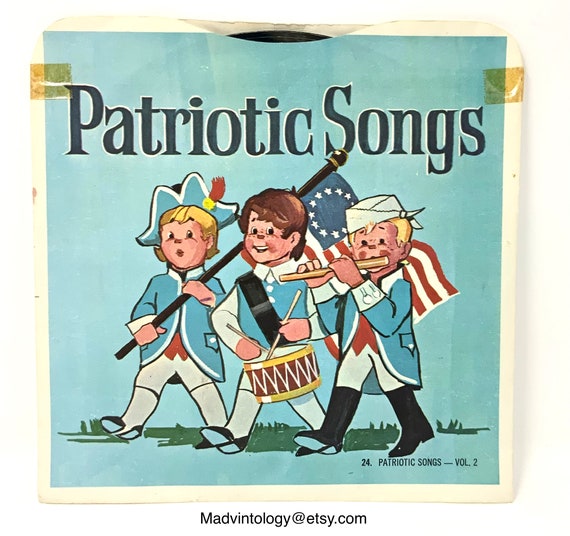This image features the cover of a vintage vinyl record with visible signs of wear such as tape marks on either side. The top of the black vinyl record peeks out from a slot in the paper cover. The cover is predominantly light blue with a greenish hue, and the title "Patriotic Songs" is prominently displayed in bold black letters at the top. Below the title, the subtitle "Volume 2" and the number "24" are noted at the bottom right corner, indicating this is the second volume in a series.

The central illustration captures a patriotic scene with three young boys marching. The boy in the center, with brown hair and no hat, is playing a drum slung over his chest with a black band. To his left is a blonde boy carrying an American flag with thirteen stars; he's dressed in a blue jacket, tricorn hat, white short pants, white socks, and black boots. On the right is another blonde boy, who has a bandage tied around his head and is playing a flute. He wears a blue jacket and white trousers. Beneath their feet is a patch of green grass, adding to the illustration’s vividness. The text "Patriotic Songs, Volume 2" and the detail "Madventology at Etsy.com" suggest the image is associated with a seller or series of historical music collections available online.

Overall, the style and setting of the cover are unmistakably patriotic, evoking a sense of historical celebration through its depiction of a lively parade scene.